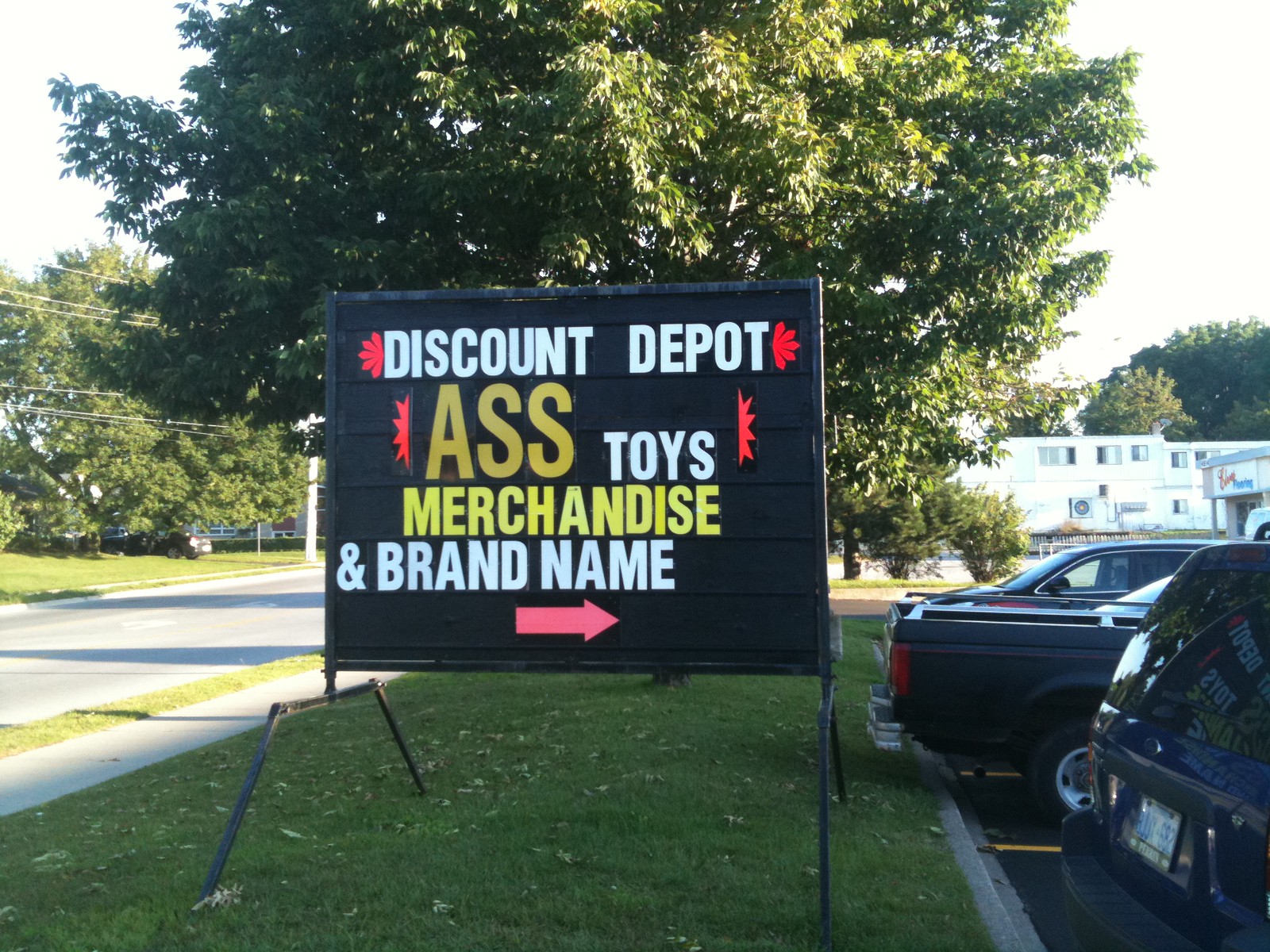The image captures a detailed scene centered on a black advertisement sign reading "Discount Depot" in white text, followed by "Ass Toys, Merchandise, and Brand Name" in a larger yellow font. A pink arrow points to the right. The sign, supported by a metal frame and two black stands, is positioned in a grassy island flanked by a sidewalk on the left and a small parking lot with three or four cars on the right. Behind the sign, a prominent green tree occupies much of the background. Further to the right, a two-story white building with multi-units, possibly containing shops, is visible along with another shop displaying indistinct red and blue signage. Additional grassy areas and trees can be seen beyond the road to the left of the sign.